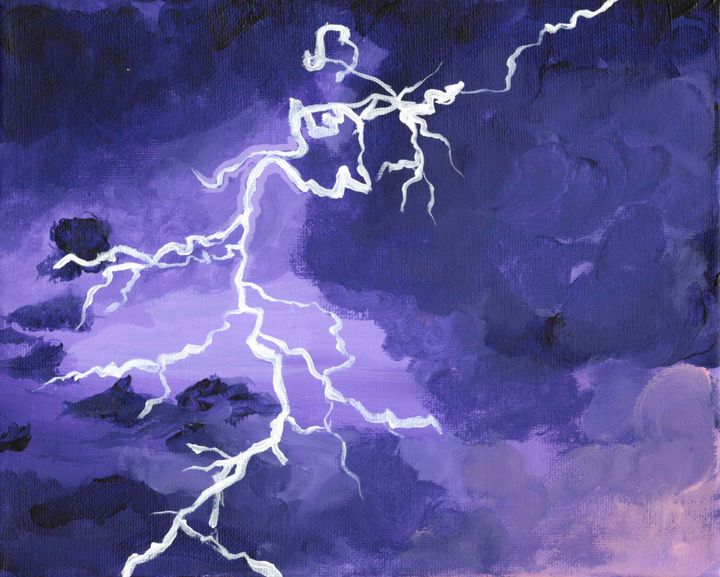The image depicts a striking painting, likely created with oil or acrylic paints on canvas, illustrating a vivid thunderstorm scene. Dominated by a stormy sky, the painting features splotchy clouds rendered in rapid, broad brush strokes. The color palette is rich with various shades of purple—ranging from deep, dark purples to muted lavenders and lilacs—interspersed with blacks to capture the brooding nature of the storm. A prominent feature is the large, spindly streak of lightning branching in multiple directions, winding down from the top right to the bottom of the image. This lightning is depicted with hurried, skillful white brush strokes, creating an effective, dynamic visual. Additional black areas within the clouds, particularly on the left side of the painting, add depth and contrast to the lighter, thicker clouds. Overall, the painting demonstrates a high level of talent and conveys the dramatic atmosphere of a thunderstorm with great detail and intensity.